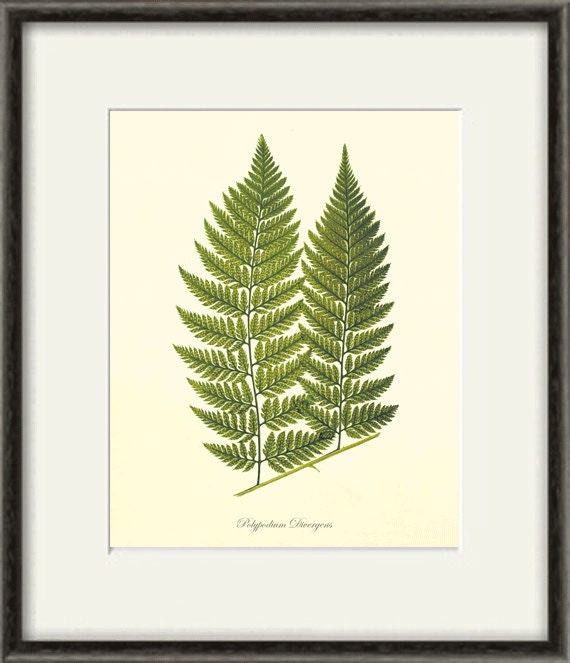The image portrays a vibrant, digitally created depiction of green ferns, meticulously framed in a black outer frame with a matted white inner border. The composition rests on a cream background, with the ferns presented diagonally, extending from the lower left to about a quarter way up the picture, where they bifurcate into two stems adorned with lush leaves. Beneath this botanical illustration, a script in black lettering – though partially obscured – appears to indicate the scientific name "Pepperdermon Dernegans," rather than the artist's signature. This detailed setup within the layered frames showcases the verdant vibrancy of the ferns in a structured yet elegant manner.